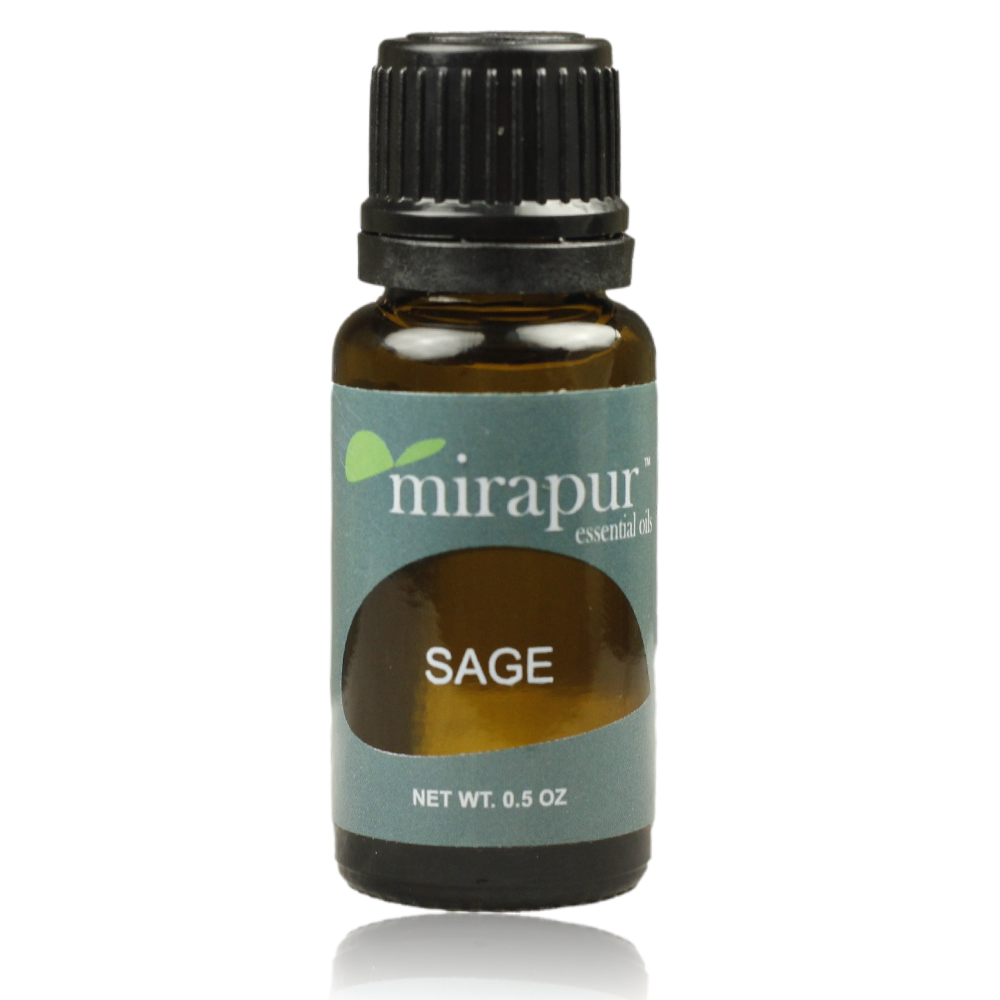The image showcases a small, half-ounce amber-colored bottle of MiraPure sage essential oil. The bottle, which features a black screw-on cap, presents a sage green label adorned with a lighter green leaf above the MiraPure logo. The white text on the label reads "MiraPure Essential Oil" and "Net Weight 0.5 ounces." An oval cutout at the center prominently displays the word "Sage." The entire design is centered, with the background blending with the turquoise hue. The bottle's shoulders reflect light, adding a subtle highlight to its overall appearance.